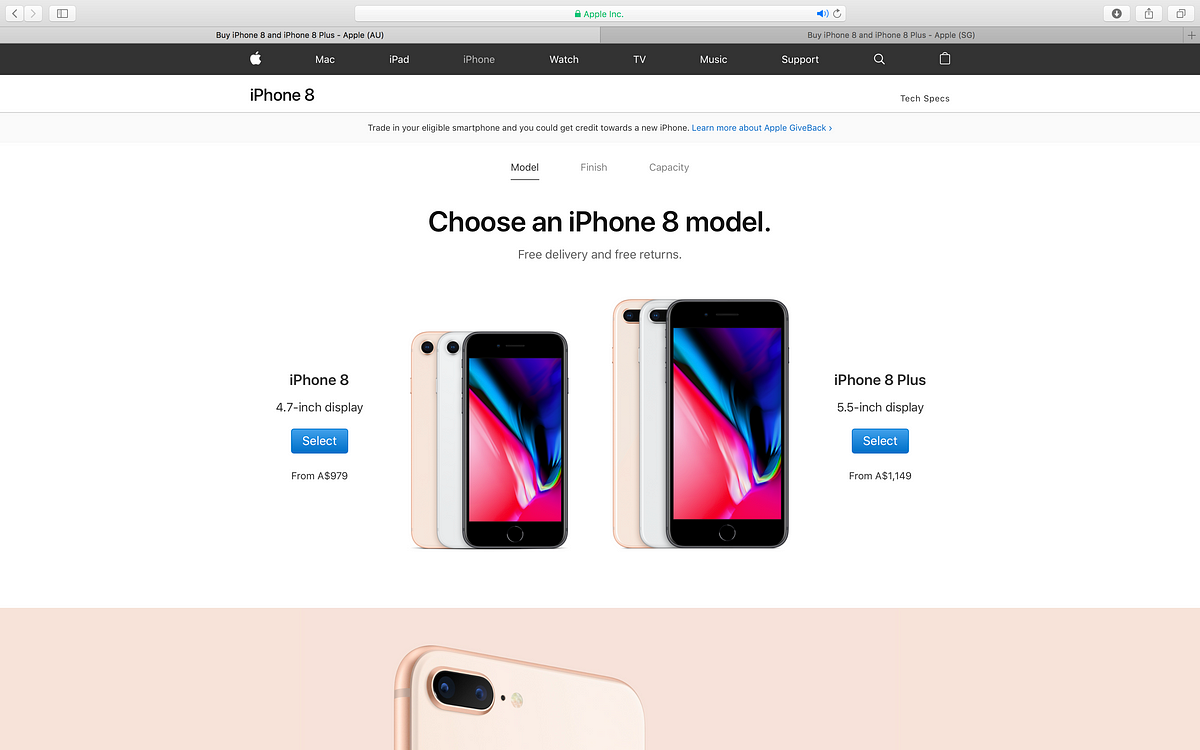A vintage promotional screenshot for the Apple iPhone 8 and iPhone 8 Plus models is displayed, showcasing the option to select between the two devices. The image highlights the differences in screen size and display information for both phones. This screenshot evidently dates back to the initial release period of the iPhone 8 lineup.